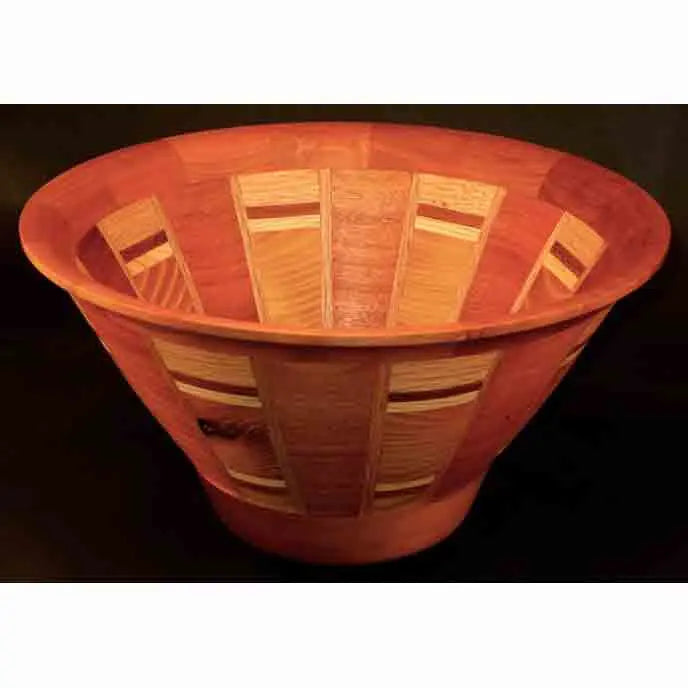The image features a meticulously crafted wooden bowl set against a solid black background. The bowl, created by Winchester Woodworks, is rectangular in shape and wider than it is tall. It has a flat base that flares out like a cone towards the top, giving it a triangular appearance rather than a completely round one. The bowl is predominantly a reddish-brown color and showcases a segmented design with multiple panels. Each panel contains slats of various shades of wood, creating a striking contrast of colors and grain patterns. The lighter wood slats range from sandy to brownish-orange, interspersed with darker brown rectangles and spots, adding to the bowl's intricate and unique design. The detailed craftsmanship is evident in the seamless assembly of these different wood pieces, making the bowl not only a functional item but also an eye-catching decorative piece. The black background accentuates the bowl's distinct colors and textures, highlighting its handmade, specialty craft nature.